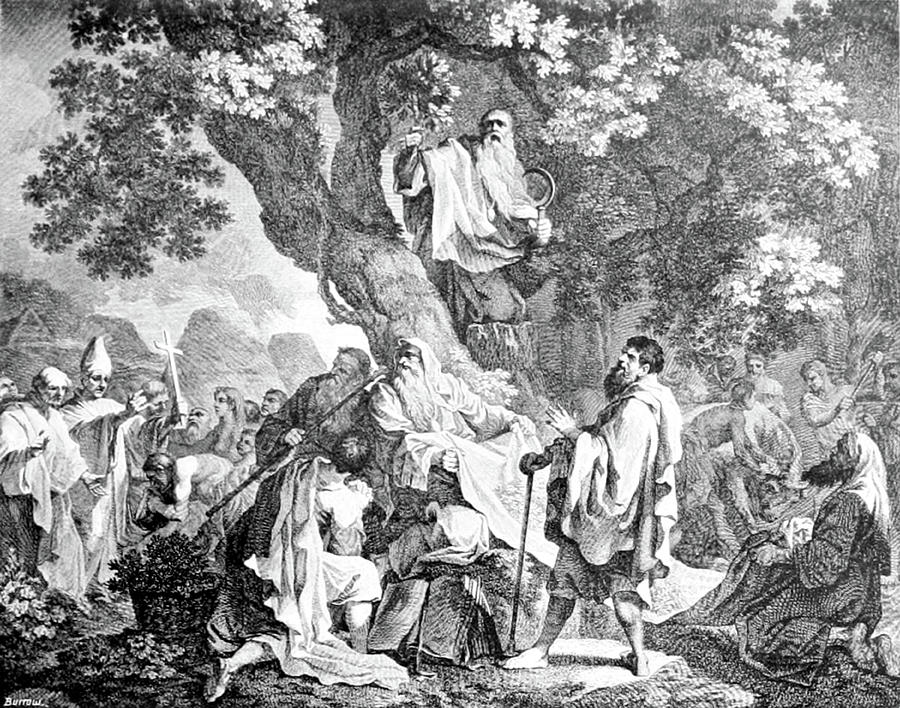This detailed black and white drawing, likely titled "Druids: The Ritual of Oak and Mistletoe," captures a significant historical or religious event. At the center, a prominent tree stands tall, its foliage artistically rendered in varying shades of gray. Perched in this tree is a man adorned in flowing robes and a long beard, clutching a sickle, bathed in sunlight. Surrounding the base of the tree, numerous figures, mostly men, dressed in draped or robe-like attire, gather in a circular formation. Many hold staffs or crosses, suggesting a ritualistic or religious gathering. Among them, a pope-like figure prominently holds a cross, while others, some prostrate, seem to be in reverence or ritual. The background is filled with more trees and figures, adding depth and complexity to the scene, all captured in intricate black, white, and gray tones, evoking an ancient and spiritual ambiance.